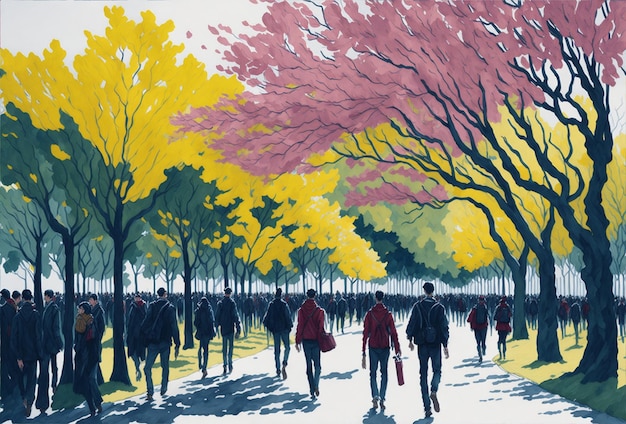This painting features a bustling city park, potentially reminiscent of a college campus, with a wide, white concrete pathway running through its center. Flanking the path are lush green grasses and a symphony of pastel-shaded trees in hues of pink, yellow, and green. The trees’ trunks and branches exhibit a mix of grayish blue and brown shades, enriching the autumnal atmosphere. The sky peeks through in a blend of white and light blue tones. The scene is animated by a large crowd, primarily depicted as faceless silhouettes in shades of gray and darker blue, adding to the sense of distance and anonymity. Most of the figures are walking away, suggesting movement towards a destination. Among the throng of young individuals, there's a notable figure of a girl in a miniskirt, possibly hinting at a nostalgic era from the late 60s or early 70s. The dense crowd and the park’s vibrant canopy create a captivating interplay between nature and human occupation, capturing the lively spirit of the setting.